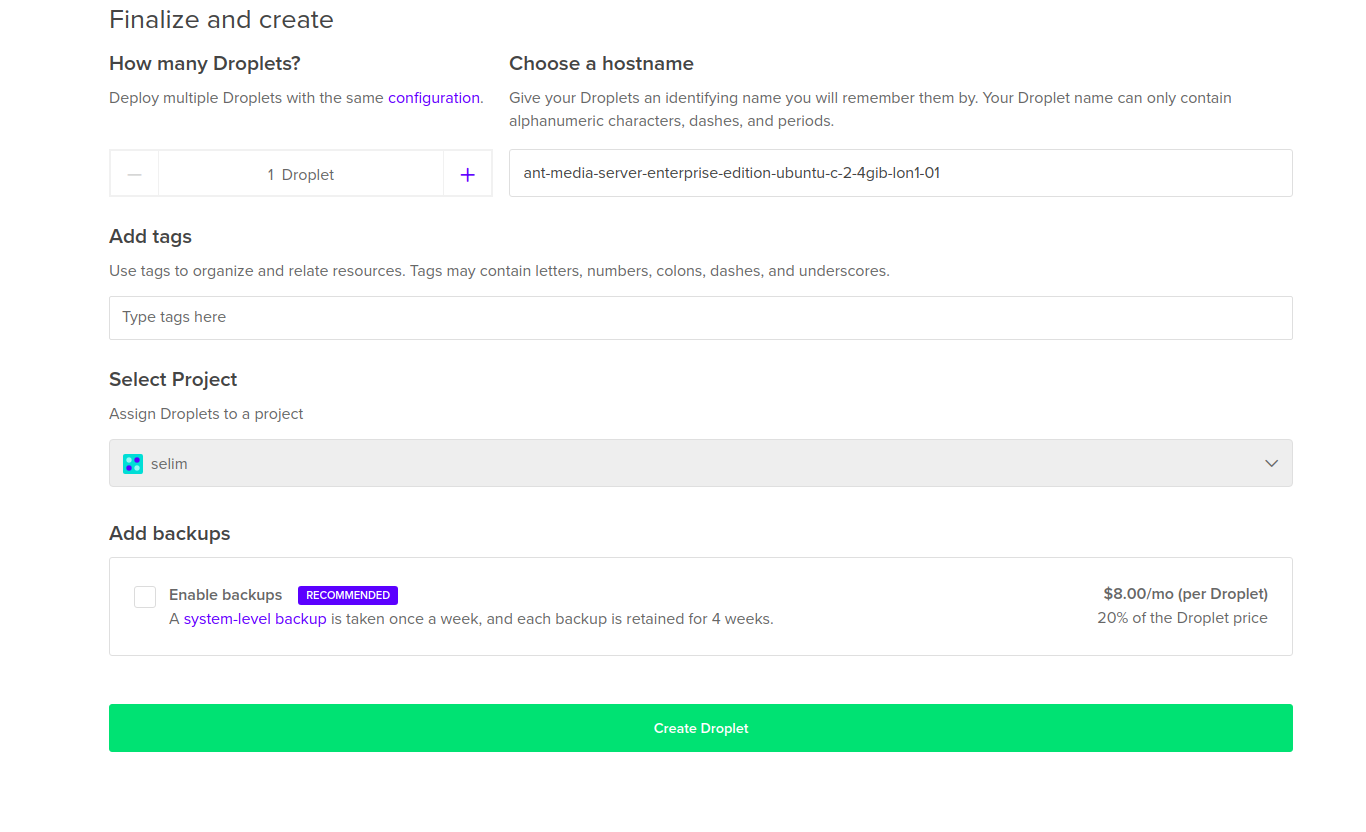The screenshot of a computer website features a clean, white background with minimal use of color. At the top left, the text reads "Finalize and create how many droplets." Just below, there is a description: "Deploy multiple droplets with the same configuration." 

On the right-hand side, there is an option labeled "Choose host name" followed by instructions: "Give your droplets an identifying name. Your droplet name can only contain alphanumeric characters, dashes, and periods."

Further down, on the left, there is a visual representation of a single droplet with a purple arrow pointing to the right. Adjacent to this, another text reads "Ant Media Server Enterprise Edition."

Below these sections, there is a prompt to "Add tags" accompanied by a text input box titled "Type tags here." Right beneath this, the option "Select project" is visible, followed by the instruction "Assign droplets to a project." Next to this section, there is a cyan blue square labeled "SELIM."

The final area at the bottom of the screenshot has an "Add backups" section. It includes a purple button that says "Enable backups (recommended)." At the very bottom of the image, a thick, dark green horizontal banner displays the text "Create Droplet."